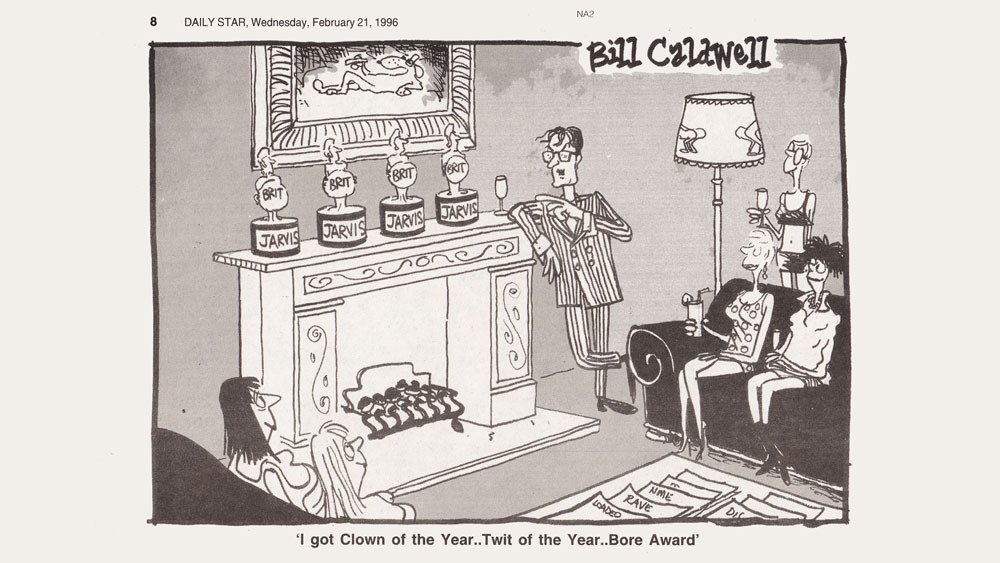This black and white cartoon panel, illustrated by Bill Caldwell and published in The Daily Star on Wednesday, February 21, 1996, resembles a classic Sunday newspaper comic strip. The scene depicts a man in a pinstripe suit, wearing glasses, standing and leaning against the mantle of a fireplace. Above the mantle, there's a whimsical painting of a dog lying on its back smoking a cigarette. Scattered across the room, mostly sitting on couches, are five women, each holding mixed drinks like mimosas and cocktails. One woman in the background is notably wearing a bikini. On the fireplace mantle, four trophies, labeled "Brit" and "Jarvis," suggest a satirical nod to the Brit Awards. The lamp beside the man features figures of naked women. The man, seemingly mansplaining, boasts, "I got Clown of the Year, Twit of the Year, Boar Award," amid a room cluttered with newspapers and surrounded by the bemused women.